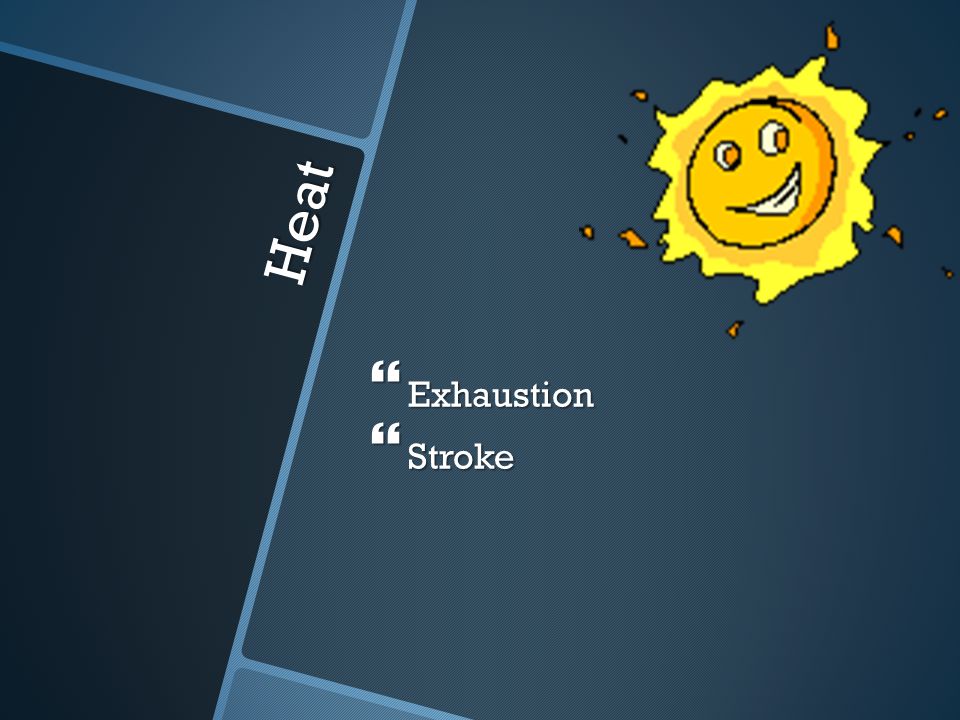The image is a color illustration combined with graphic design and typography, displayed in a landscape orientation. The background consists of four angled rectangles divided by light blue grid lines, in varying shades of dark blue and teal. The leftmost rectangle, colored in dark navy blue, features the word "heat" in white text, rotated approximately 30 degrees counterclockwise to align with the rectangle's edge. In the upper right corner, there's a bold yellow sun graphic with a smiling face, characterized by orange eyes, an open mouth, and yellow flames laced with orange on the outer edges. Near the center of the image, below the sun graphic, are two lines of white text. The first line reads "exhaustion" in quotation marks, and the second line reads "stroke," also in quotation marks. The overall style blends vivid color illustration with typographic elements to convey a likely public service message about heat-related illnesses.